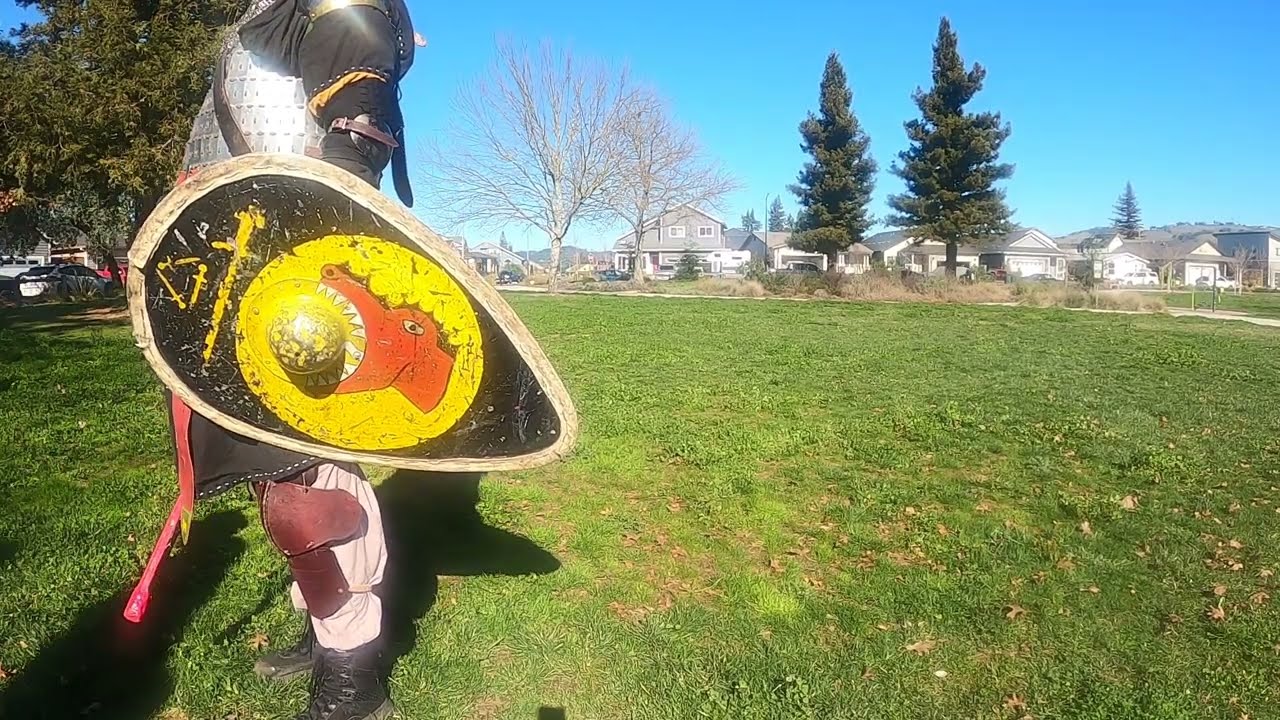In the image, a person dressed as a medieval knight stands prominently in a grassy field, which has patches of both green and brown grass, indicating a well-used space. The individual is positioned on the left side of the image, with their left profile visible, though their head is cut off by the top of the picture. They are adorned in a metal chestplate with a leather belt crossing it, red kneecaps, and leather shin guards, suggesting a detailed reenactor's costume or a renaissance fair actor.

The knight holds a teardrop-shaped shield in their left hand, which appears well-worn and battle-scarred. The shield has a striking design featuring a red dragon's head with its mouth open, a yellow symbol, and an image resembling a sword and a meteorite within a bordered wooden frame. Their outfit includes a gold rope tied around the arm, shiny silky cloth details, and black shoes.

In the background, the scene transitions from the grassy field to a suburban setting, with a line of residential homes stretching across the horizon. The houses vary in size, with a notably large gray house flanked by smaller homes. The background also features tall pine trees and bare deciduous trees, suggesting a winter setting. A pathway breaks the field, and towards the left side of the image, you can spot cars and additional foliage. The bright blue sky and sunny conditions emphasize the vividness of the outdoor setting.